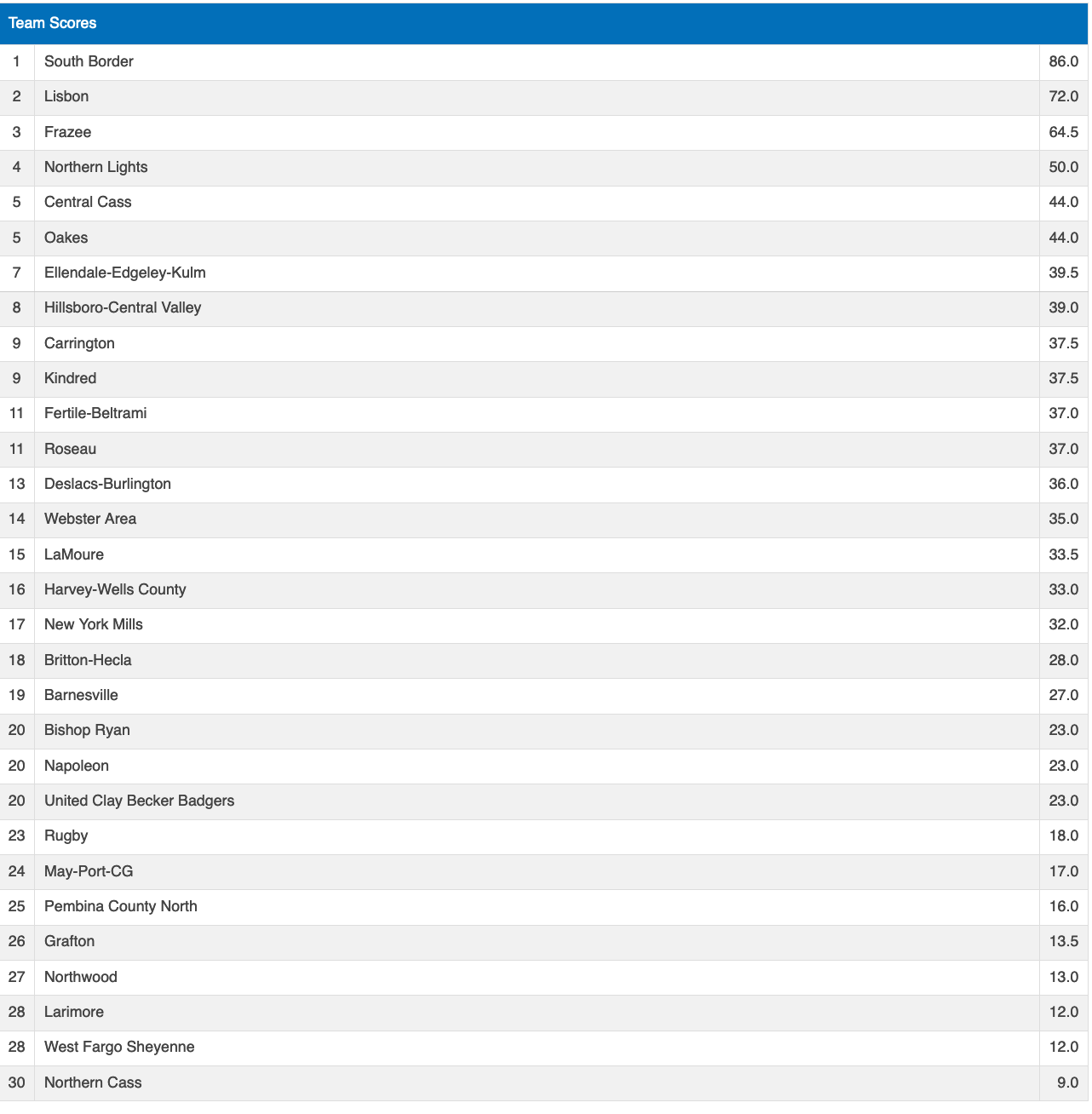This image captures a screen showing a list of team scores on a website or document. At the very top, a blue banner displays the text "Team Scores" in white font. Below the banner, a ranking of 30 teams is presented, each with their respective scores displayed on the far right side of the screen. The teams and their scores are as follows:

1. South Border - 86
2. Lisbon - 72
3. Frazee - 64.5
4. Northern Lights - 50
5. Central Cass - 44
5. Oakes - 44
7. Ellendale/Edgeley/Kulm - 39.5
8. Hillsboro/Central Valley - 39
9. Carrington - 37.5
9. Kindred - 37.5
11. Fertile-Beltrami - 37
11. Roseau - 37
13. Des Lacs-Burlington - 36
14. Webster Area - 35
15. LaMoure - 33.5
16. Harvey/Wells County - 33
17. New York Mills - 32
18. Britton-Hecla - 28
19. Barnesville - 27
20. Bishop Ryan - 23
20. Napoleon - 23
20. United Clay Becker Badgers - 23
23. Rugby - 18
24. May-Port CG - 17
25. Pembina County North - 16
26. Grafton - 13.5
27. Northwood - 13
28. Larimore - 12
28. West Fargo/Cheyenne - 12
30. Northern Cass - 9